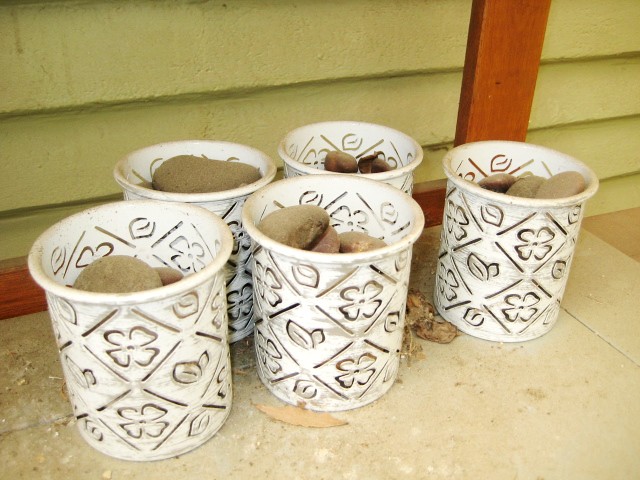This photograph features five white, off-white containers placed next to a wooden structure with light lime green vinyl siding and contrasting orange-red trim. The containers, which resemble pint-sized ice cream cups, are adorned with intricately cut-out designs forming alternating diamond patterns. Within each diamond, either a simple four-petaled flower or a pair of diagonal leaves is delicately carved. The containers, showing signs of dirt and debris, rest on a large-tiled concrete or stone surface, presumably an entryway or porch, with noticeable grouting lines.

Each container is filled to the brim with smooth, light to medium brown fist-sized rocks and stones, likely to be used for decorative or functional purposes such as in walkways or as paperweights. Scattered around the base of the containers are various pieces of debris, including leaves and what appears to be part of a paper towel. Additionally, a red piece of vinyl or wood, possibly a chair, is visible near the containers, adding to the scene's visual interest. The lighting illuminates the details effectively, highlighting both the containers’ decorative patterns and the texture of the stones.